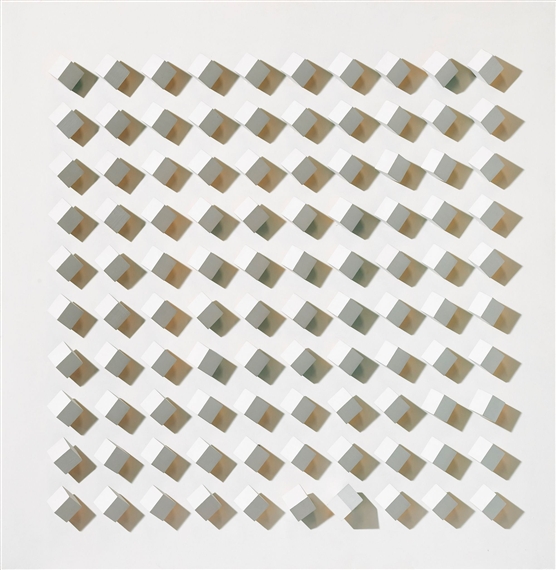The image, titled *Atmosphére Chromoplastique, North Degrees 109, 1963* by artist Luis Tomasello, features an abstract composition with a light gray background. This square format painting prominently displays a grid of 3D cubes, each meticulously arranged in a symmetric pattern. The grid comprises 10 rows horizontally and 10 vertically, forming a total of 100 cubes. Each cube exhibits slight variations in shades of gray and beige, enhancing the three-dimensional effect and giving depth to the overall arrangement. Notably, on the very bottom row, one of the cubes stands out, being tilted on its side, breaking the otherwise uniform grid. The overall design exudes an artistic exploration of light and shadow, emphasizing geometric precision and abstract form.